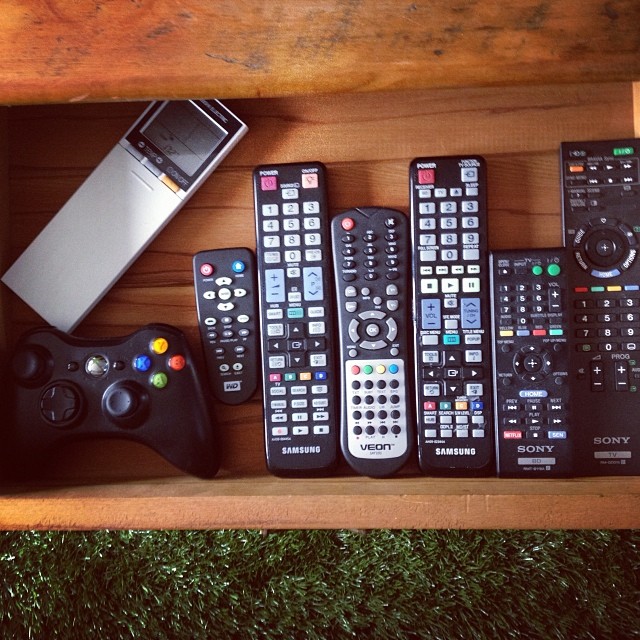This detailed color photograph captures a top-down view of an open wooden drawer extending outward from a dresser with a medium brown finish. The drawer, which is positioned on short, likely artificial grass, contains several electronic control devices meticulously arranged. On the left side of the drawer is a black Xbox controller, featuring the classic colored buttons: blue X, yellow Y, green A, and red B. Directly above the Xbox controller sits a white temperature controller, distinguished by a small screen at the top and a cover that conceals its buttons. To the right of these devices are six television remotes, lined up vertically. Among them are two Sony remotes, two Samsung remotes, a Vyond remote, and an unbranded one, each showcasing a multitude of buttons in various colors. The collection of controllers and remotes in this photograph points to a well-organized storage of outdated or spare control devices in a wooden drawer, captured against the contrasting greenery of the artificial grass below.